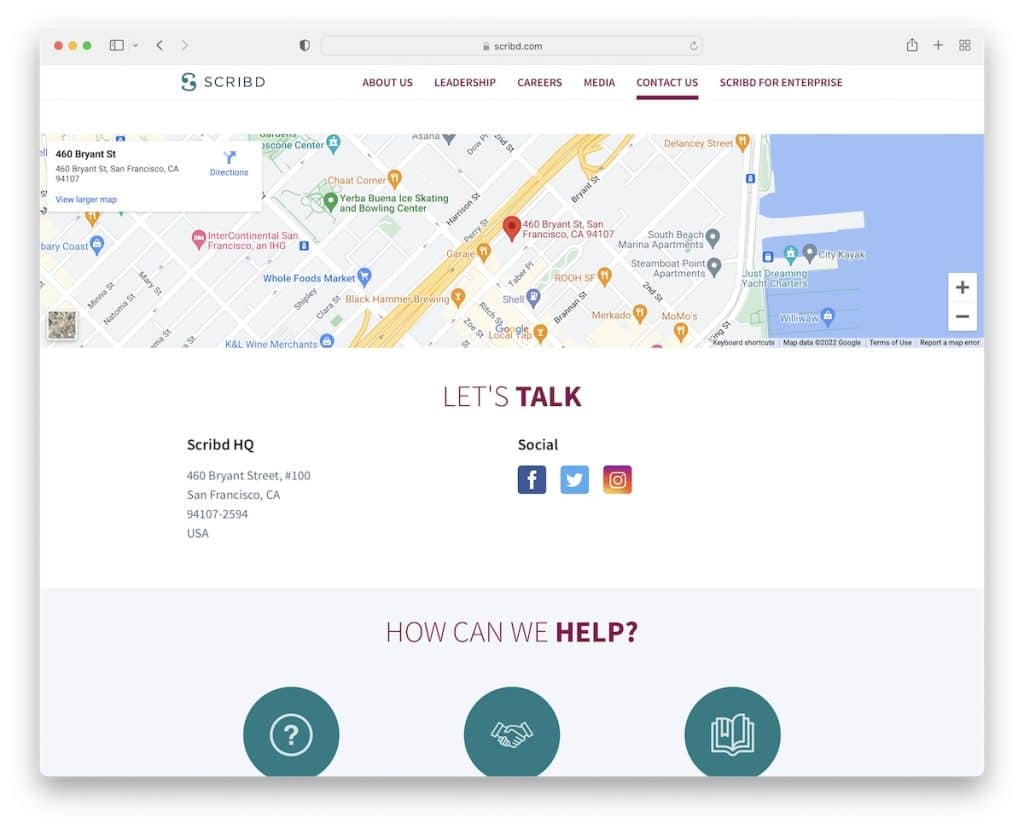This screen capture appears to be of a webpage, likely from scribed.com, featuring a detailed map interface. At the very top, there's a gray navigation bar displaying a trio of circular buttons in red, gold, and green. Following these buttons, additional icons in gray include back and forward arrows, a shield symbol, and a URL bar secured with a padlock, showcasing the address “scribed.com.” Adjacent to this are icons for refresh, a box, a plus sign, and a grid of four squares.

Beneath this bar, a white banner features the text “Scribed” in black, accompanied by a small teal logo. Situated in a plum color are navigation links for “About Us,” “Leadership,” “Careers,” "Media," and “Contact Us,” with “Contact Us” underlined. Another section reads “Scribed for Enterprise.”

The main content area showcases a view similar to Google Maps, pinpointing the address as "460 Bryant Street, San Francisco, California 94107." A white pop-up box on the map lists this address, along with options to “View larger map” and get “Directions” highlighted by a blue arrow. The map itself is populated with various location pins: restaurants marked with orange icons, a business with a green pin, one with a pink pin, and several shopping spots using blue pins. A red pin marks the exact location of 460 Bryant Street.

Towards the bottom of the screen, a plum-colored section states “Let's Talk,” featuring social media icons for Facebook, Twitter, and Instagram. The location is identified again as “Scribed HQ” with the same Bryant Street address. Another plum section poses the question, "How can we help?" followed by three teal icons indicating different types of support: a question mark, a handshake, and a book, each in white.